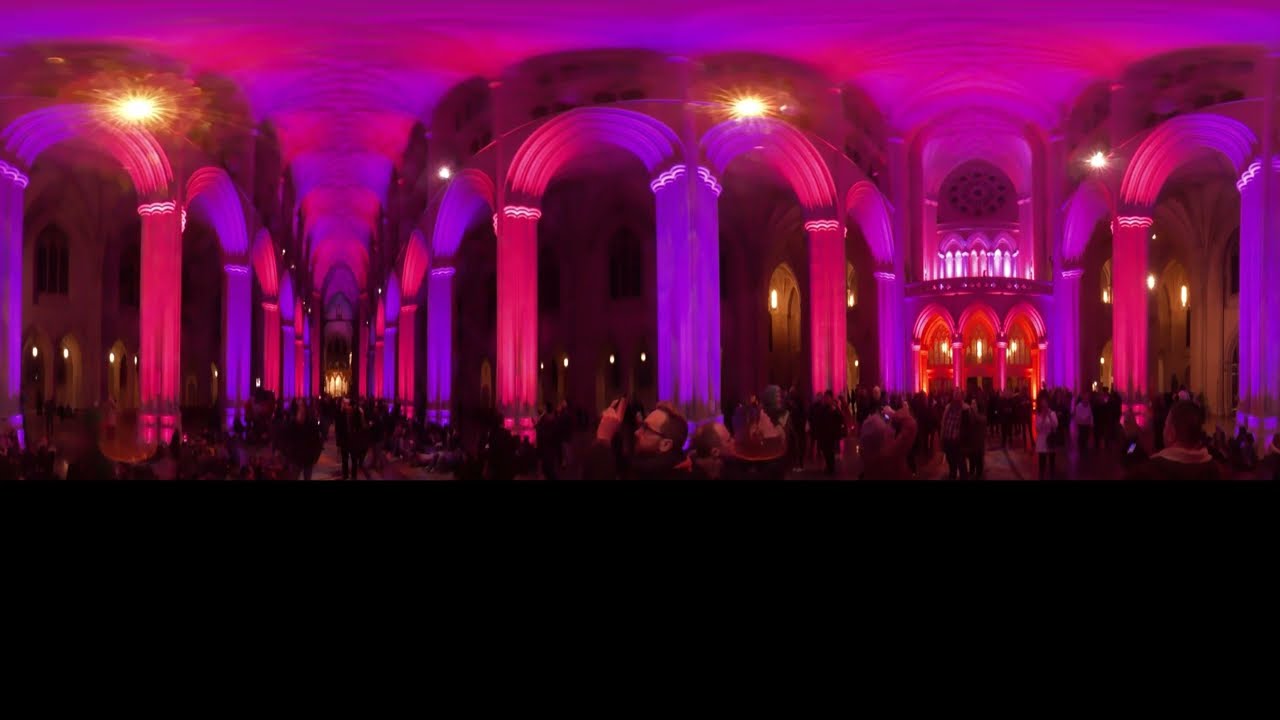The photo captures the exterior of a grand, large building adorned with numerous archways, all illuminated in a vibrant red hue. The building appears monumental, with over twenty arches stretching from the left to the right, leading to a smaller fountain structure before continuing further. A balcony holds prominence on the right side, under which three archways glow in pink light. Above the balcony, there's a distinctive half-circular window composed of triangular shapes.

In front of the building, there is a noticeable crowd of people milling about, though their features are indistinct due to the dim lighting, which casts their clothing mostly in dark hues. There are brighter lights attached to some of the pillars—specifically positioned on the left, center, and right. In the backdrop, additional buildings form a silhouette with a dark brown coloration, amplified by the lack of direct lighting.

Dominating the foreground is the prominent face of a man with a bald head, beard, and mustache, which stands out sharply against the darker, red-lit environment of the image. Overall, the scene is dark yet vividly accented by the dramatic red and pink lighting, enhancing the structure's architectural features and the bustling activity beneath it.